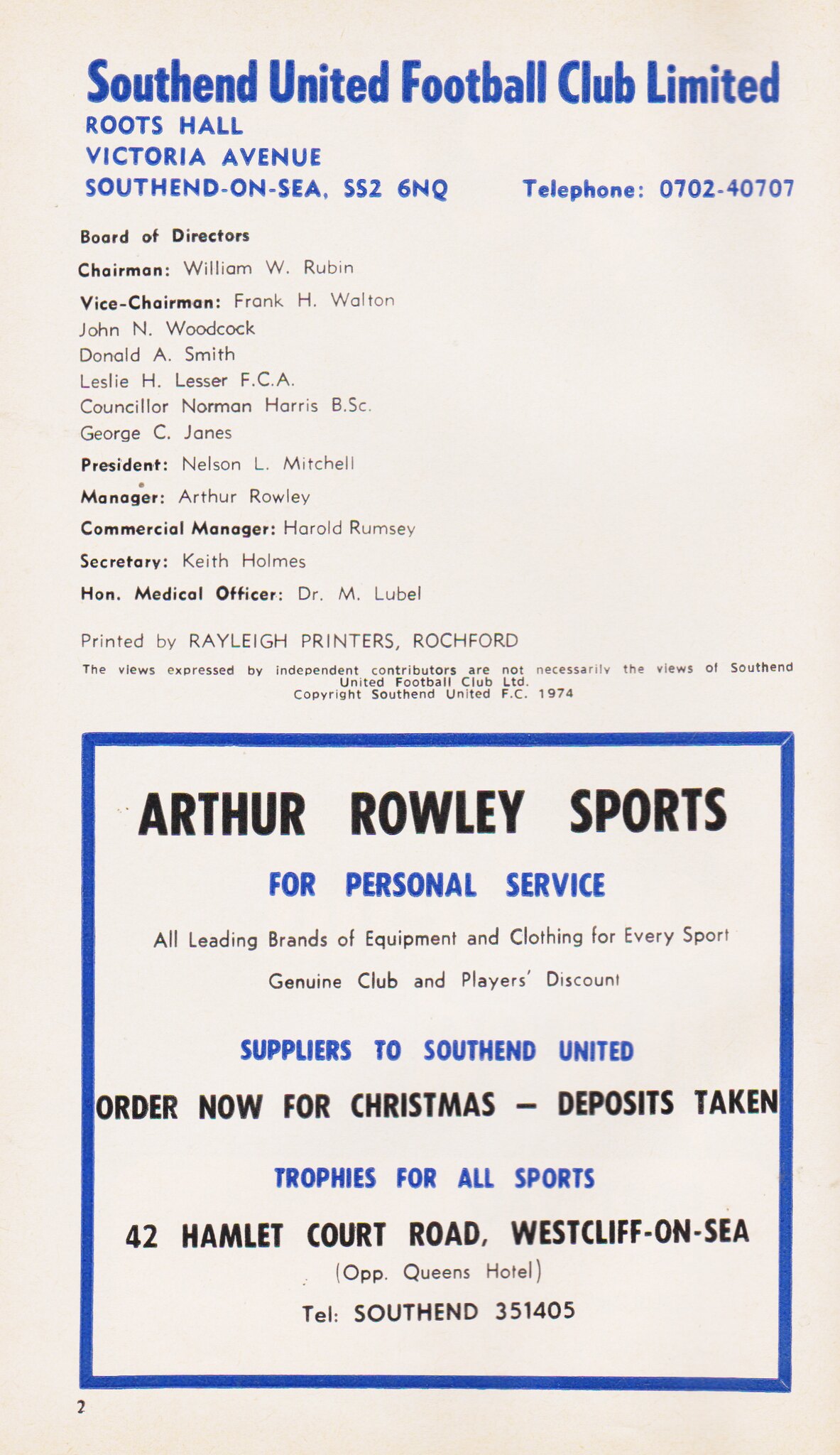This image from a South End United Football Club Limited booklet features detailed club information against a light off-white background. The header, written in blue ink, reads: "South End United Football Club Limited, Rootes Hall, Victoria Avenue, South End on C, SS2 6NQ, Telephone 0702-40707." Below, in black text, a list is provided detailing the Board of Directors: Chairman William W. Rubin, Vice Chairman Frank H. Walton, with members John N. Woodcock, Donna Rae Smith, Leslie H. Lesser, Counselor Norman Harris, and George C. Jones. Further roles include President Nelson L. Mitchell, Manager Arthur Riley, Commercial Manager Harold Rumsey, Secretary Keith Holmes, and Medical Officer Dr. M. Lubell. Printing credits are given to Raleigh Printers, Rocheford. At the bottom, bordered by a blue square, an advertisement for Arthur Rowley Sports highlights their personal service and extensive range of sports equipment and clothing. They offer genuine club and player discounts, are suppliers to South End United, and accommodate Christmas orders with deposits accepted. Additionally, they provide trophies for all sports. The shop is located at 42 Hamlet Court Road, Westcliff-on-Sea, with a contact number of South End 351405.